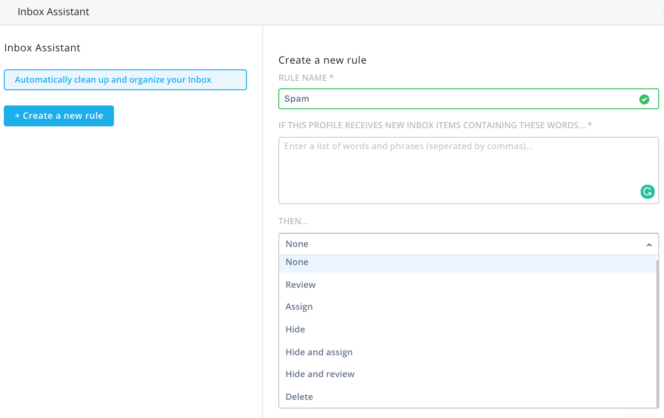The image depicts the interface of a software named Inbox Assistant. At the top of the screen, there is a light gray horizontal bar with black text on the left side that reads "Inbox Assistant". Below this bar, the screen is divided into two sections.

The left section features the heading "Inbox Assistant", beneath which there is a blue box containing the text "Automatically Clean Up and Organize Your Inbox". Below this text, there is a solid blue button with the label "Create a New Rule".

The right section is dedicated to rule creation. At the top, it prompts the user with "Create a New Rule" and provides a field to name the rule. Below this, there is a description that reads, "If this profile receives new inbox items containing these words", followed by a text entry area where users can input specific words or phrases. Further down, it contains a section labeled "Then...", which presents multiple action options: None, Review, Assign, Hide, Hide and Assign, Hide and Review, or Delete.

Users can formulate a rule by combining a rule name, specified keywords, and one of the listed actions. This customized rule will then be employed by the Inbox Assistant to manage the incoming messages accordingly.